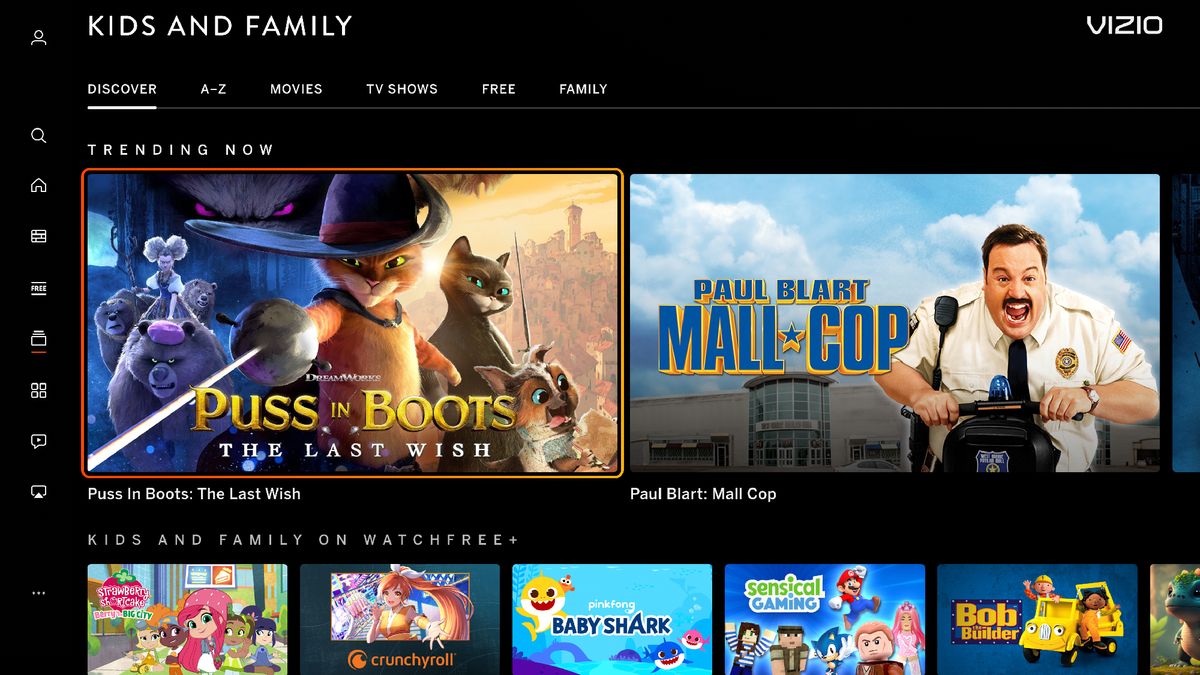This is a screenshot from the Vizio app designed for Vizio flat-screen televisions. In the top left corner, the "Kids and Family" section is prominently displayed. The app's interface features a vertical black menu on the left side with several icons, including a profile icon, search function, home button, and various other options which are not clearly identifiable. 

Below the "Kids and Family" heading, there is a horizontal menu with tabs labeled "Discover," "A to Z," "Movies," "TV Shows," "Free," and "Family." Directly beneath this menu, the "Trending" section is highlighted. 

The first item in the "Trending" section is a large, vibrant graphic for "Puss in Boots: The Last Wish," showcasing the titular cat in a hat and sword, accompanied by other characters, castles, and mythical elements—indicative of the movie's DreamWorks animation and its popular status. 

To the right of this, another prominent rectangle features "Paul Blart: Mall Cop," depicting the main character, played by Kevin James, riding a scooter in his security uniform, caught mid-yell, with a mall setting in the background.

Further down, sections labeled "Kids," "Family," and "Watch Free" display various cartoon thumbnails including "Baby Shark," among others. There are about six options visible at the bottom, though the text underneath them is partially cut off, making them unreadable. The overall layout of the app is reminiscent of popular streaming services like Netflix.